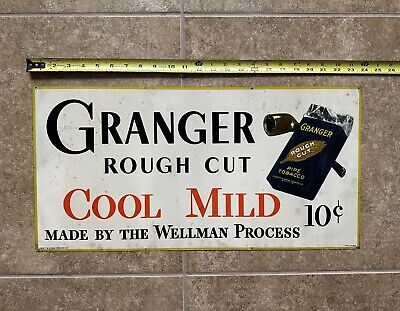In this photograph, a rectangular, predominantly white poster is affixed to a wall made of brown-gray square tiles. The poster prominently features the word "Granger" in large font, followed by "rough cut" and "cool mild" in red text, "made by the Wellman process," and "10 cent." To the right of the text is an illustration depicting a black cigarette-like box labeled "Granger" with a brown leaf incorporating the words "rough cut" and a smoking pipe positioned behind the box. Above the poster, a yellow tape measure with centimeter and inch markings measures its width.